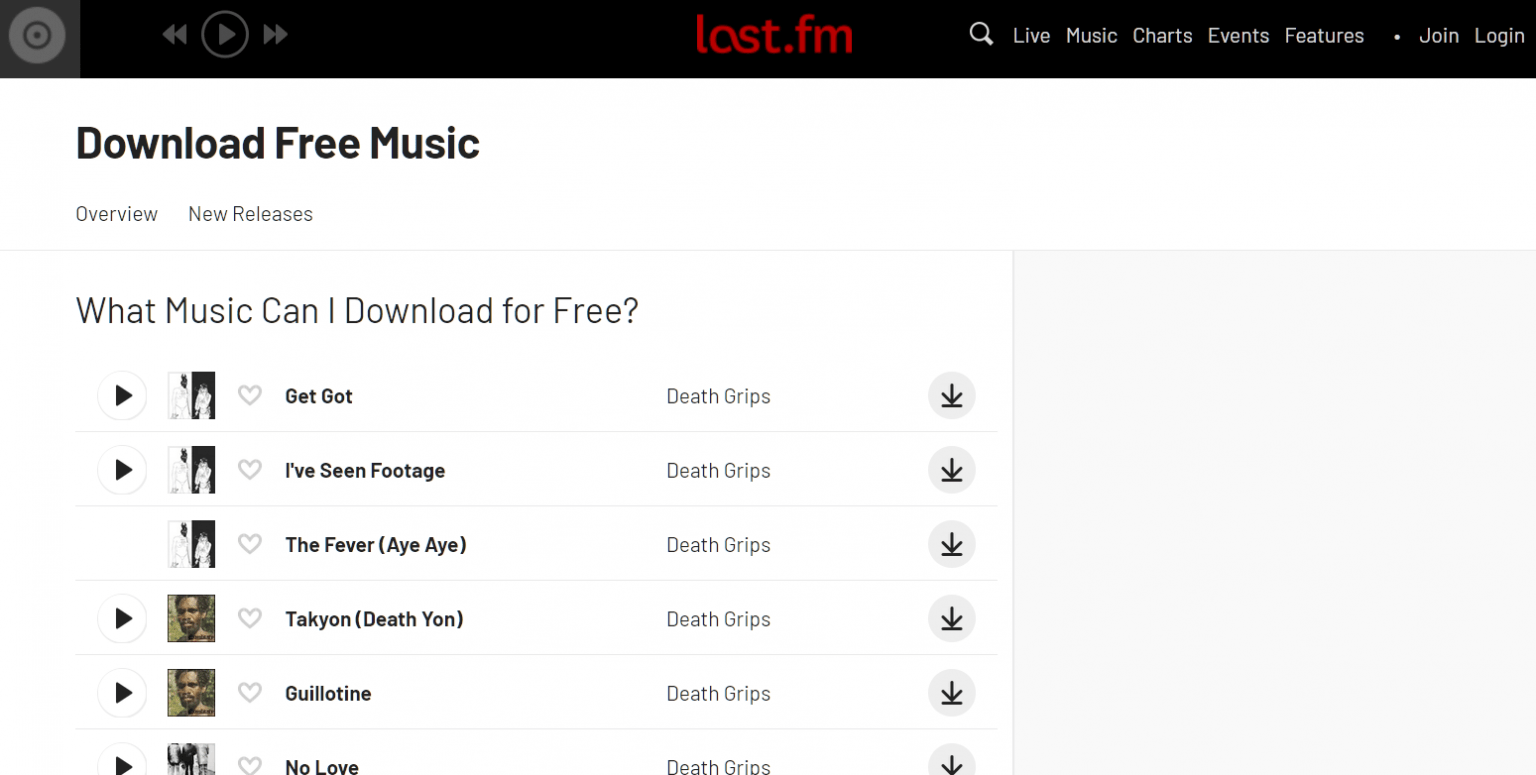The image depicts a detailed interface of a music streaming platform. At the top, there is a grey disc followed by a grey square. To the left, there’s a black left arrow button, a play button, and a right arrow button. Below these, there's a distinct red section labeled "last.fm" accompanied by a magnifying glass (indicating a search function), and various tabs titled "music," "charts," "events," and "features." There's also a red circle with the options "join" and "login."

In black text, the phrase "download free music" is prominently displayed. Underneath this, tabs such as "overview," "new releases," and "what music can I download for free?" are listed. Scattered throughout the interface are multiple play buttons and a few down arrows.

The music listed includes tracks by Death Grips, such as "I've Seen Footage," "The Fever," "Attack Yawn," "Death Yawn," and "Guillotine." Each track is accompanied by a heart icon and a play button. Users can interact with the platform through play buttons, arrows for navigation, and heart icons for favorites. In the background, there are grey down arrows and varied lines, creating a structured yet complex layout.